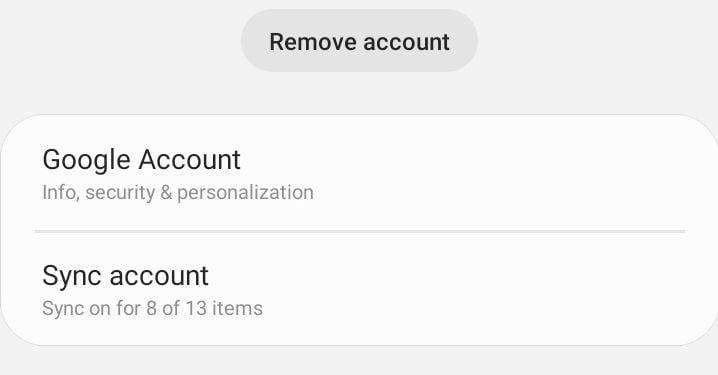This is a cropped and enlarged screenshot depicting the "Remove Account" section within Google settings. The image is primarily set against a grey background. At the top center of the screenshot, a lighter grey button labeled "Remove Account" in bold black font is prominently visible. Directly beneath this button, there's a sizeable white box divided horizontally by a grey line. 

In the upper portion of the white box, on the left-hand side, the label "Google Account" appears in bold black font, accompanied by smaller grey text stating, "Info, Security, and Personalization." Below the aforementioned grey line, the section titled "Sync Account" is displayed in bold black lettering. Underneath it, in a smaller grey font, it reads, "Sync on for 8 of 13 items."

The right edge of the white box extends out of the frame, indicating that the screenshot does not fully capture the entire width of this section. The image provides a detailed view of the key elements within this part of the settings page, focusing on the "Remove Account" option and the relevant information regarding account synchronization, all framed within a grey contextual background.